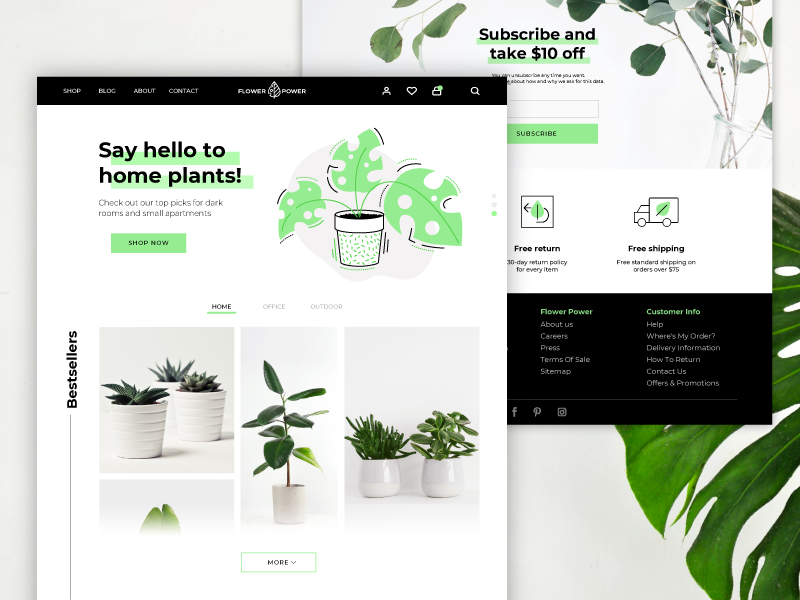**Descriptive Caption:**

Explore the inviting world of "Hello Home Plants," a comprehensive platform for purchasing a diverse range of plants. The site features a clean and functional layout, with a prominent subscription offer highlighted in green, promising a $10 discount on first-time subscriptions. This offer is showcased in an overlapping box on the top right side of the screen. Adjacent to it, there are various images of plants with long, slender stems and leaves, creating an appealing visual atmosphere. 

Below this section, visitors can enter their email to subscribe, accompanied by information on data privacy. Navigational steps are provided, although partially obscured by a pop-up box promoting a 30-day return policy, symbolized by a curved left arrow with a leaf. Another enticing feature is the free standard shipping on orders over $75, represented by an icon of a moving truck embellished with a leaf.

Further elements on the page include "Flower Power," a section with links to "About Us," "Careers," "Press," "Terms of Sale," and "Site Map," all under a green heading. To the right, customer support options are readily available, including order tracking, delivery information, return instructions, contact details, and offers.

The site also boasts a sales section prominently marked with a green-highlighted "Sale" banner and a drawing of a plant with three leaves. Users can easily navigate to shopping categories like Home, Office, Outdoor, or explore more plants through clickable buttons. Additional functionalities include a blog, contact page, user login, favorites section, and an intuitive cart and search option, all designed to enhance the shopping experience.